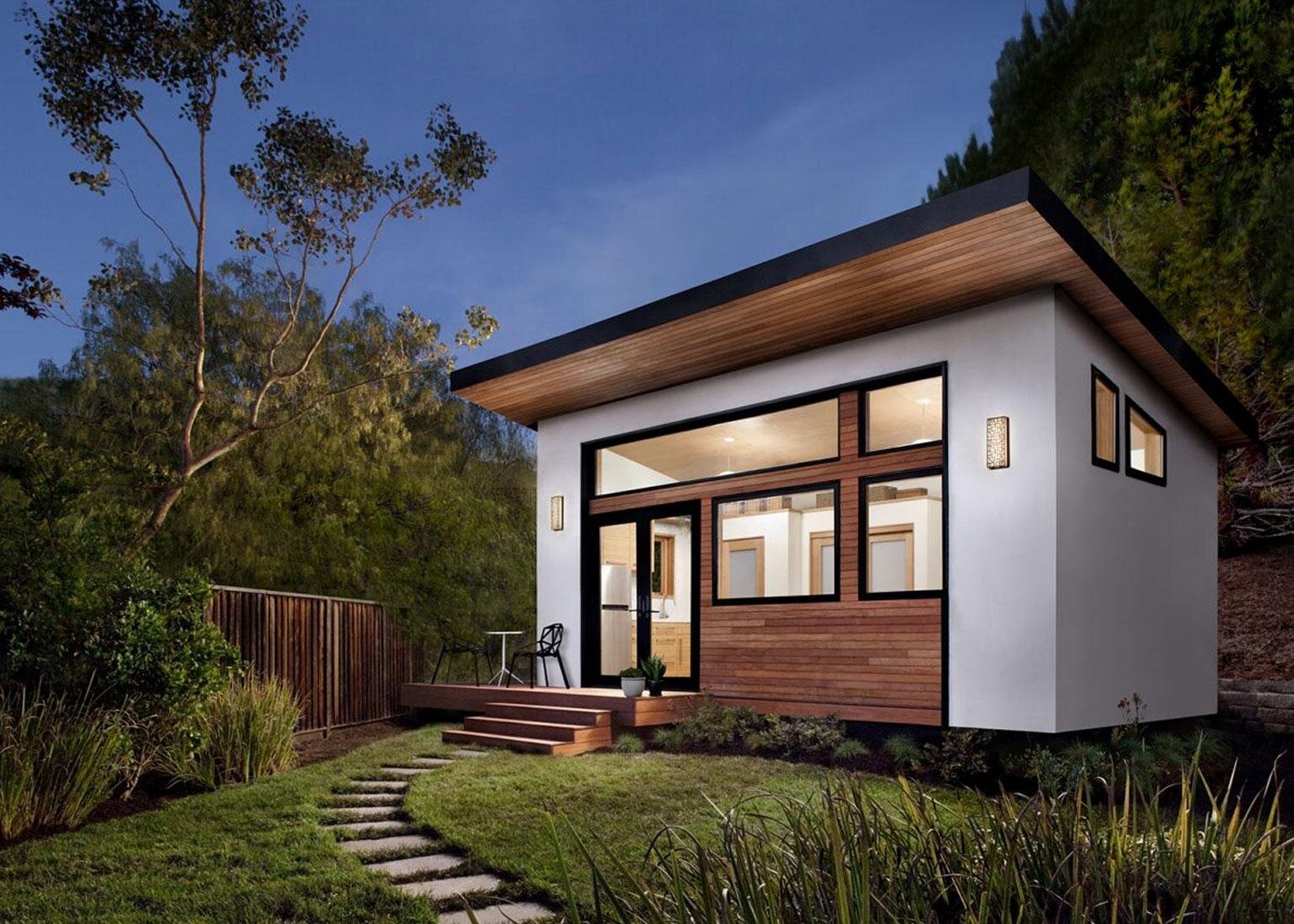The image depicts a newly built, modern tiny house positioned just right of center with striking white walls and a distinctive flat roof. The house, lit from within, reveals glimpses of a cream-colored, well-lit kitchen area featuring a silver refrigerator, a brown dresser, and a kitchen counter visible through its extensive glass windows and double glass doors.

The front of the house almost entirely features glass elements including a long window on the top left, a small window to its right, and two smaller windows beside the front double doors. Wooden elements are noticeable around the house, with brown wood framing some windows and the underside of the roof displaying a wooden texture.

The exterior includes three wooden steps leading up to a small wooden platform in front of the glass doors, where potted plants and a small white pedestal table with a chair are placed. A curved stone pathway winds through the green lawn from the front entrance, flanked by shrubs and taller grass. A wooden fence lies adjacent to brown wood-paneled areas below the windows and close to nature, giving a sense of seclusion surrounded by trees and bushes. The blue sky stretches above, with large trees in the top left and hilly masses of foliage on the right, enhancing the scenic, tranquil setting of this tiny, modern home.